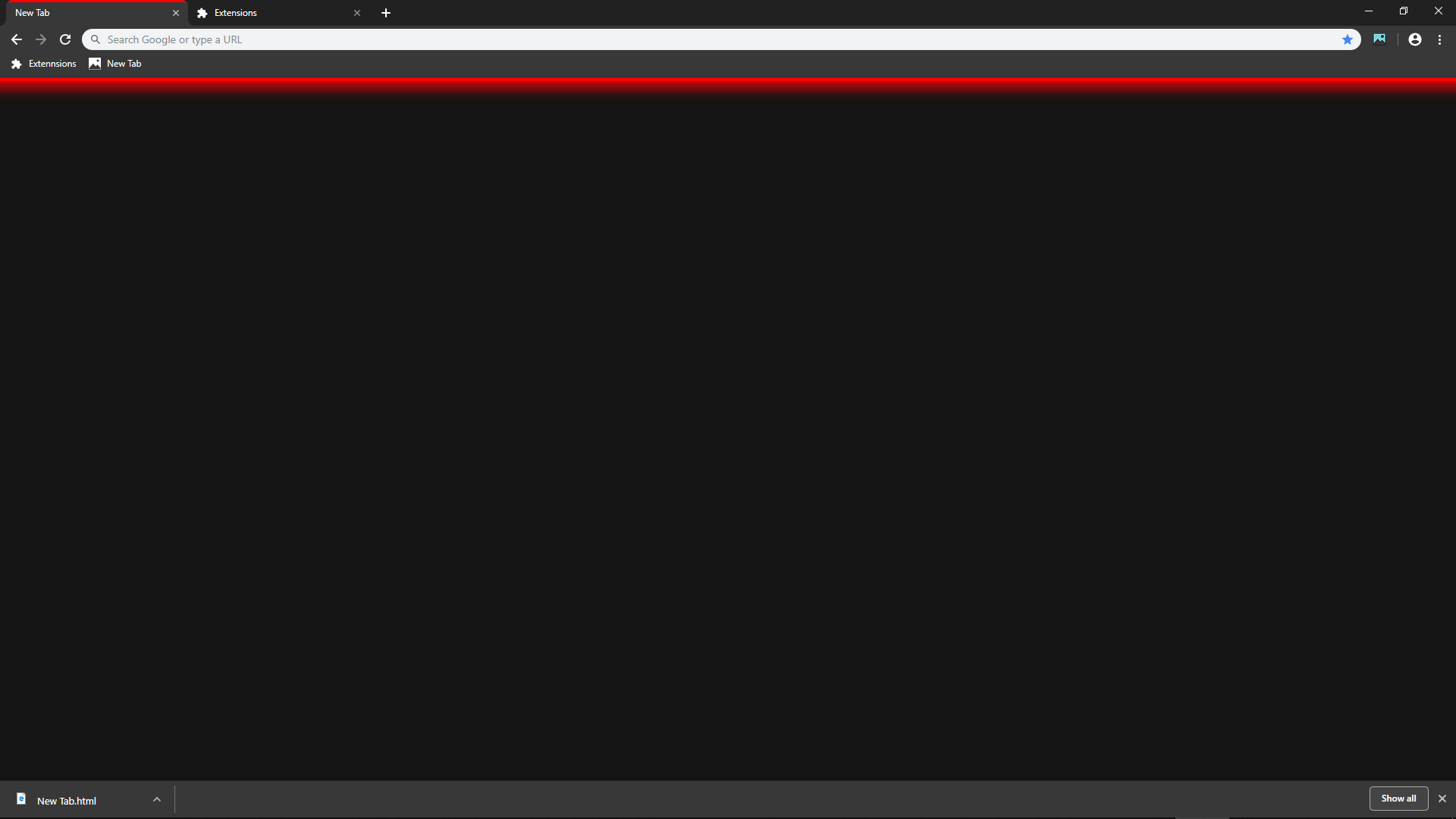The image showcases a dark-themed webpage. At the top of the page, there is a prominent search bar with the placeholder text "Search Google or type a URL." On the upper-left, a gray bar is visible. The browser interface itself is black with a left-pointing arrow. A striking red bar spans the entire width from left to right at the top of the page. Below this red bar, the background turns pitch black, devoid of any elements. A series of icons are aligned on the top right and bottom right of the screen. In the lower portion, white text accompanied by a small symbol is present, albeit barely legible due to its minuscule size. The overall layout suggests it is viewed on a computer, with the top and bottom sections extending further than the vertical sides. The deep black background makes the red bar the most colorful and noticeable element on the page.